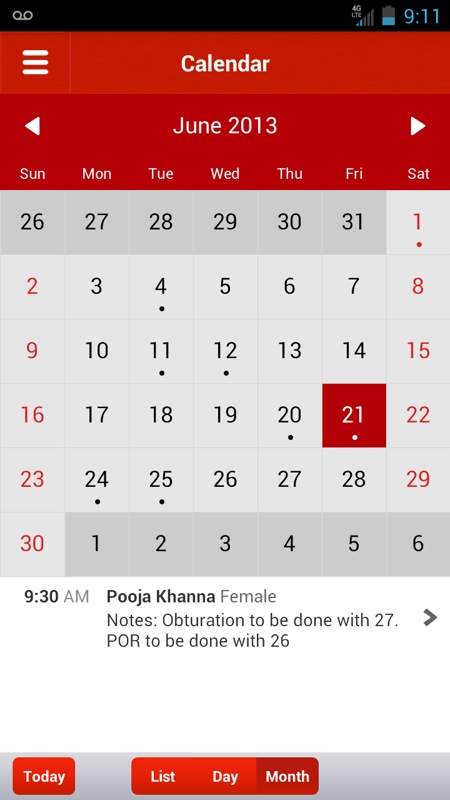This image is a screenshot taken from an Android smartphone in June 2013. The interface features an older Android version, identifiable by the blue color scheme in the data icons, typically seen in Ice Cream Sandwich or Jelly Bean versions. In the upper right-hand corner, the phone displays a 4G LTE connection with two out of five bars for signal strength. The battery level icon shows approximately 40% charge. The time displayed is 9:11, without an AM or PM designation. In the upper left-hand corner, there is a voice recorder icon indicating that a voice message is present.

The main focus of the screenshot is the Calendar app, characterized by a red and white color scheme. The selected day is Friday, June 21st, 2013. An event is scheduled for 9:30 AM with details including the name Pooja Khanna and a note regarding "obituation to be done with 27, POR to be done with 26." The interface displays options for viewing by day, list, or month, with the month view currently selected.